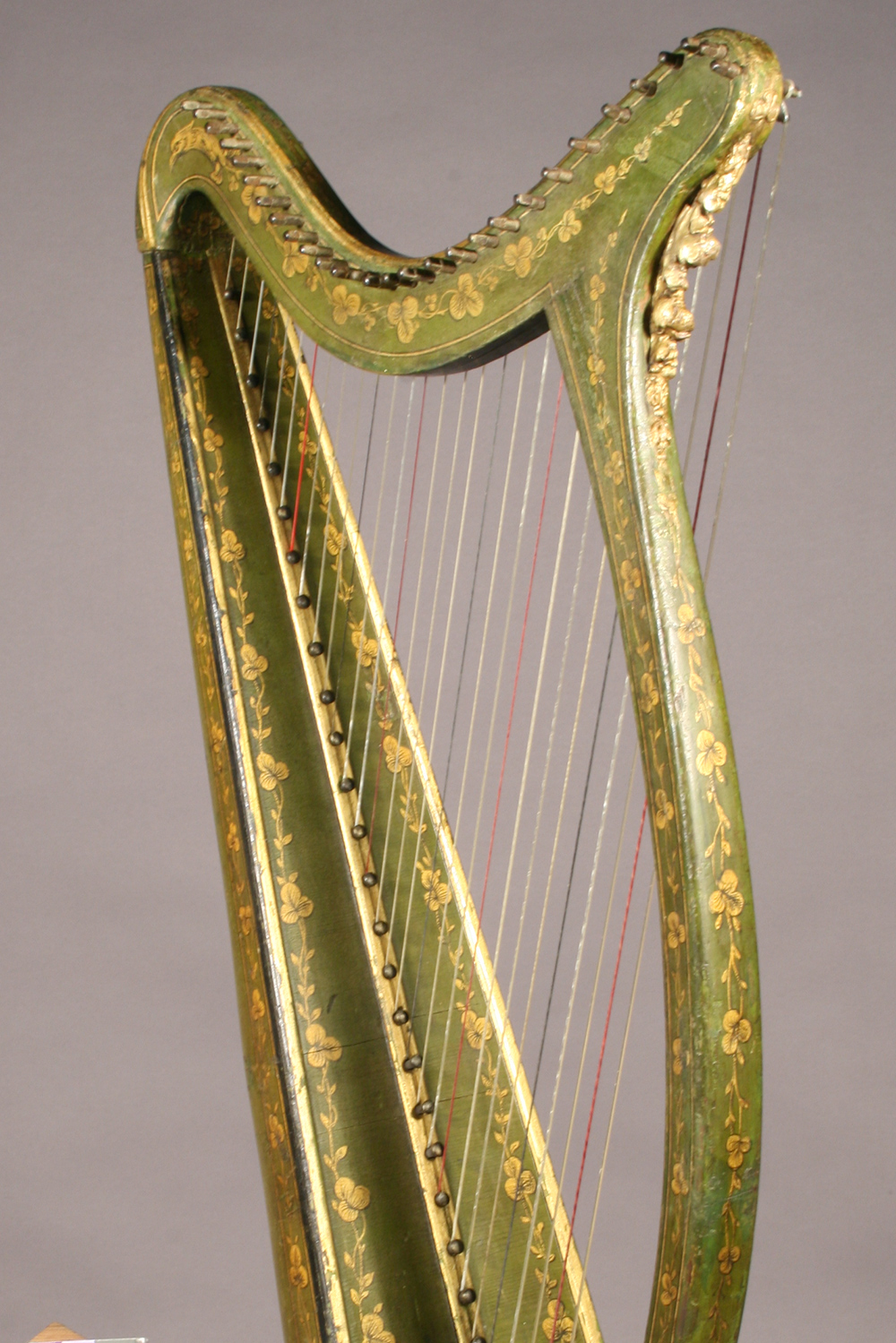This image appears to be a hyper-realistic rendering, likely an AI-generated depiction of a vintage harp. The harp itself is predominantly gold in color, adorned with intricate floral patterns that give it an antique and delicate appearance. Despite being hyper-realistic, some details suggest it's a rendering, such as the strings, which are inaccurately colored in shades of red, yellow, white, blue, and possibly green. These strings do not align correctly, raising questions about their functionality if the harp were real. The background is a plain, tan or gray color, providing a neutral backdrop that emphasizes the harp's ornate design and colorful strings. The harp features gold or brown tuning knobs along the top, consistent with its intricate craftsmanship. The image is very close-up, with no people or additional objects in the frame, focusing solely on the harp's detailed and artistic attributes.